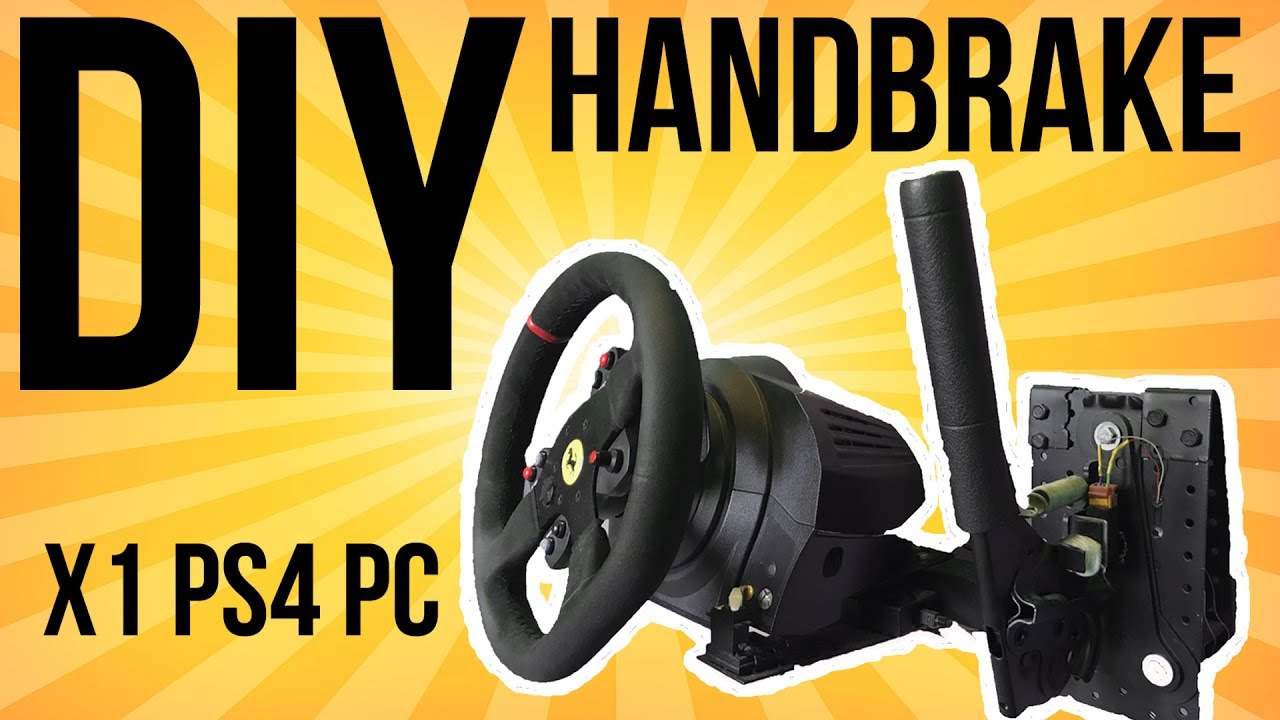The poster, set against a vivid yellow background, showcases an advertisement for a black handbrake positioned prominently towards the center-right of the image. Accompanying the handbrake is a sleek, black steering wheel adorned with the iconic Ferrari logo in black and yellow. The handbrake is depicted in an upright position, emphasized by bold black text on the left side of the poster reading "DIY HAND BRAKE." Further large text at the bottom left corner states "X1 PS4 PC," indicating its compatibility with multiple gaming platforms. Surrounding the centerpiece are intricate circuits and mechanical parts, adding a technical dimension to the visual. Red and green wires are visible, enhancing the detailed gaming aesthetic of the setting.